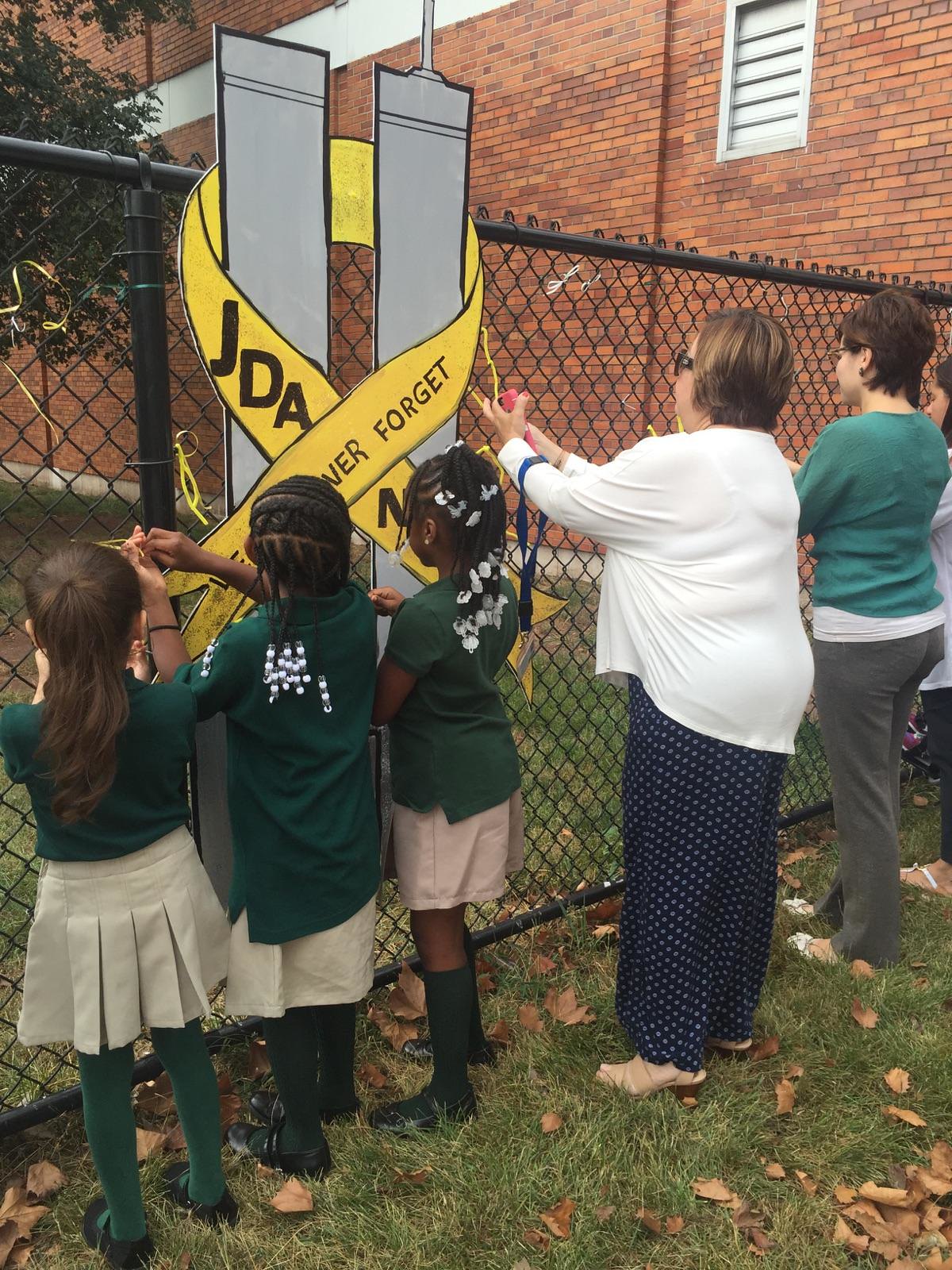In the photograph, a group of six people - three adult women and three young girls - are seen fastening a large cardboard sign onto a tall black cyclone fence, which serves as a poignant 9-11 memorial. The three little girls, likely in elementary school, stand to the left and are dressed in uniforms consisting of green shirts with khaki skirts and long socks; two have black hair and one has brownish hair. The three adult women, interspersed on the right, wear white and green jackets paired with blue, grey, and black pants, respectively. The memorial sign they are hanging depicts the Twin Towers wrapped in a large yellow ribbon with the words "JDA" and "Never Forget" in black text. Behind the fence, a tall red brick building with white trim can be seen, along with grass and trees in the distance. The image captures a moment of community effort and remembrance as the group works together to erect this tribute.